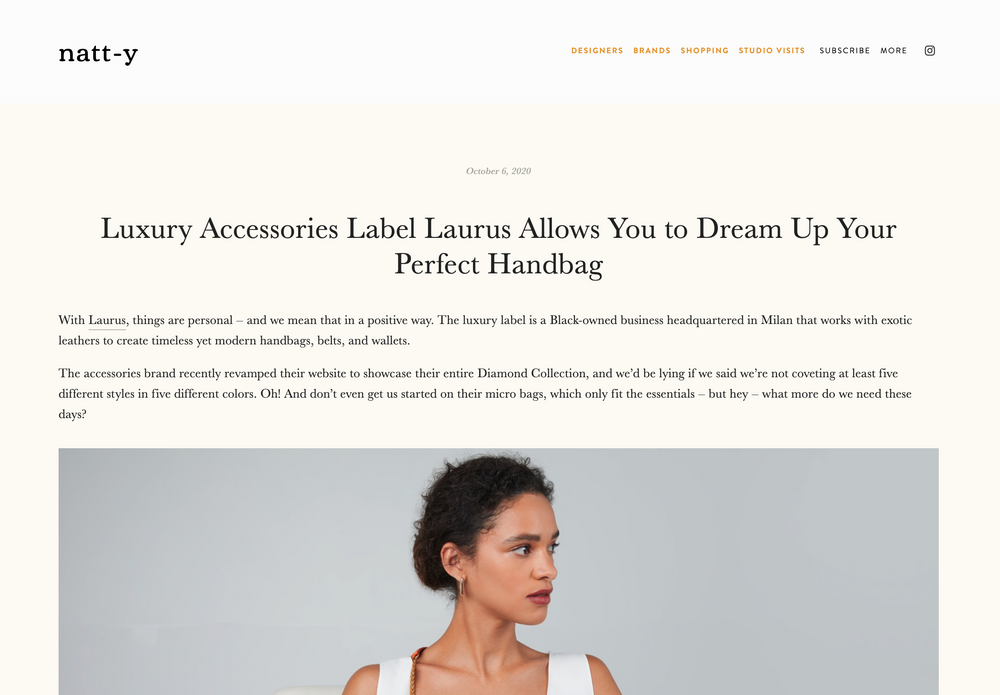This is a screenshot of an online article from the website "NATT-Y," dated October 6, 2020. The article is titled "Luxury Accessories Label Lazarus Allows You to Dream Up Your Perfect Handbag," highlighting the brand Lazarus, a black-owned business headquartered in Milan. The text elaborates that Lazarus focuses on creating timeless yet modern handbags, belts, and wallets using exotic leathers. Recently, Lazarus revamped their website to feature their complete diamond collection, and the article gushes over the desirable designs and micro bags that fit just the essentials. Accompanying the text is a photograph of a young black woman looking to her left, showing only her head and shoulders. She wears a white top, short black hair, earrings, and possibly a necklace, with beads visible on the left side of the image. At the page's top are clickable tabs for designers, brands, shopping, studio visits, subscribe, and more, along with an Instagram icon.